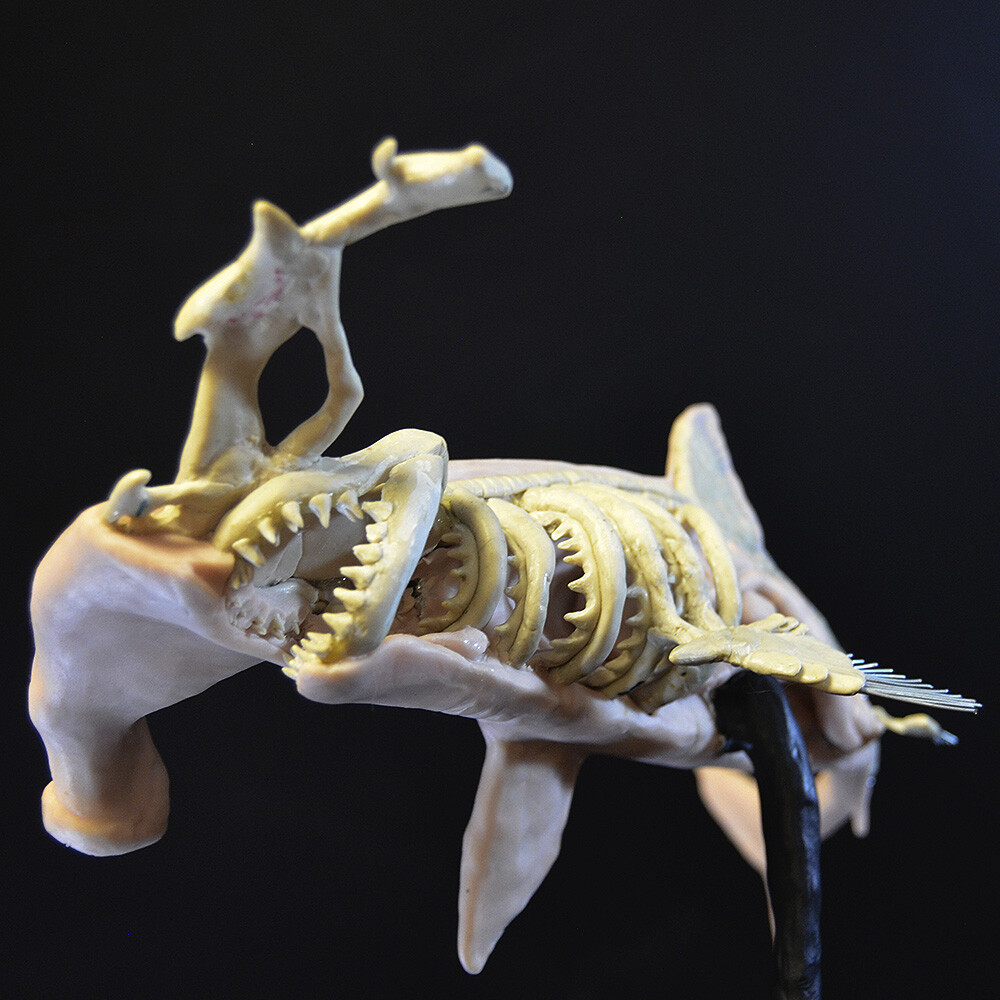The image depicts a meticulously crafted model of what appears to be a hammerhead shark, set against a stark black background for dramatic effect. The model is divided vertically, showcasing a dual representation: the left side features detailed recreations of the shark's flesh and skin in a pink hue, while the right side reveals the intricate yellow bone structure underneath. This half-and-half design emphasizes the juxtaposition between the external and internal anatomical features. The hammerhead’s distinctive T-shaped head and wide-set eyes are prominently displayed, with the left side of the head cut away to expose the inner skeletal framework. The mouth is filled with rows of sharp teeth, a feature that runs the length of the skeletal structure visible within the model. Fins and a tail are present, partially exposed to highlight both the muscle and bone elements. The entire model is mounted on a small black pole, adding to its museum-like presentation.